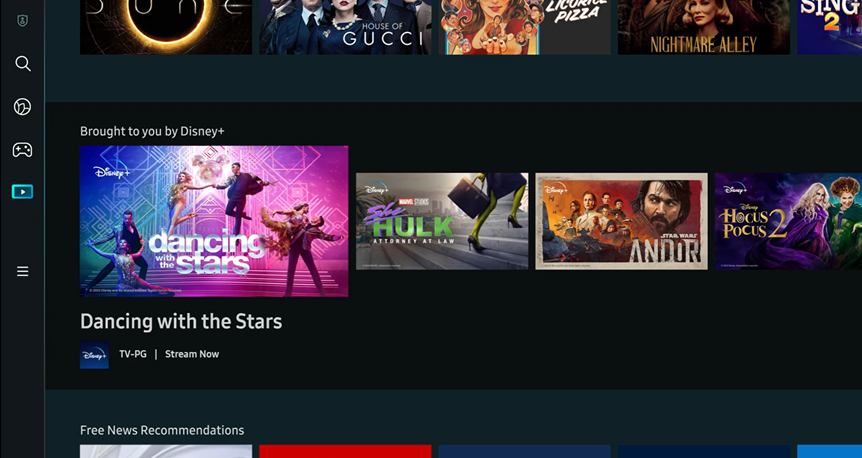The screenshot appears to capture a streaming interface, likely from Disney+. On the left side of the screen, a vertical navigation bar displays several icons: a profile icon, a search icon, a globe or world icon, a game controller icon, and a play icon. Below these, there is a hamburger menu icon.

Central to the image, there is a banner with the text "Brought to you by Disney+" in white. Beneath this banner, a row of icons for different shows is visible. The highlighted show is "Dancing with the Stars," along with its rating (TV-PG) and a "Stream Now" button. Adjacent to it are icons for "She-Hulk," "Andor," and the movie "Hocus Pocus 2."

Below the highlighted show, there's mention of "Free News Recommendations," with partially visible news shows on the lower left edge of the screen. Above the Disney+ row, another row showcases icons of non-Disney movies, barely identifiable but including titles such as "Dune," "House of Gucci," "Licorice Pizza," "Nightmare Alley," and "Sing 2."

The entire interface is set against a predominantly black or dark gray background, with minimal extraneous design elements, keeping the focus on the content displayed.